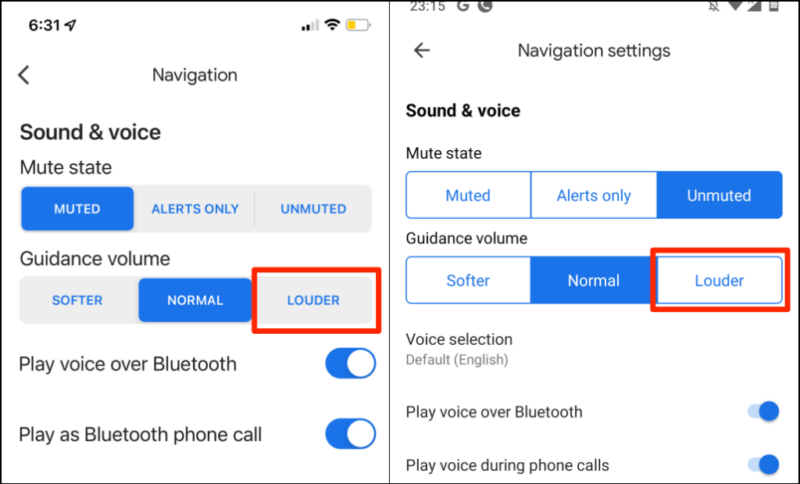The image comprises two horizontally aligned screenshots of a mobile phone, displaying settings for a navigation app. Both screenshots focus on adjustable options related to sound and connectivity within the navigation settings. The options listed include "Sound and Voice," "Mute State," "Guidance Volume," "Play Voice Over Bluetooth," and others. Users can customize how navigation audio behaves, such as deciding the volume level of navigation prompts, muting or setting alerts, and choosing whether to play voice commands over Bluetooth devices.

Each screenshot displays various selections, indicated by highlighted blue boxes that denote the active option. For instance, options like "Muted," "Alerts Only," and "Unmuted" are visible, with specific choices highlighted. Additionally, both images show toggle switches for options like "Play Voice Over Bluetooth." These toggles are depicted with a white circle inside a blue oval; the circle’s position on the right indicates the toggle is active. All four visible toggles—two in each screenshot—are in the 'On' position.

Furthermore, each screenshot contains status information at the top: the current time is displayed on the left, while indicators for battery life, data connection, and wireless network signal are visible on the right. These status indicators provide context about the phone’s operational status at the time the screenshots were taken.